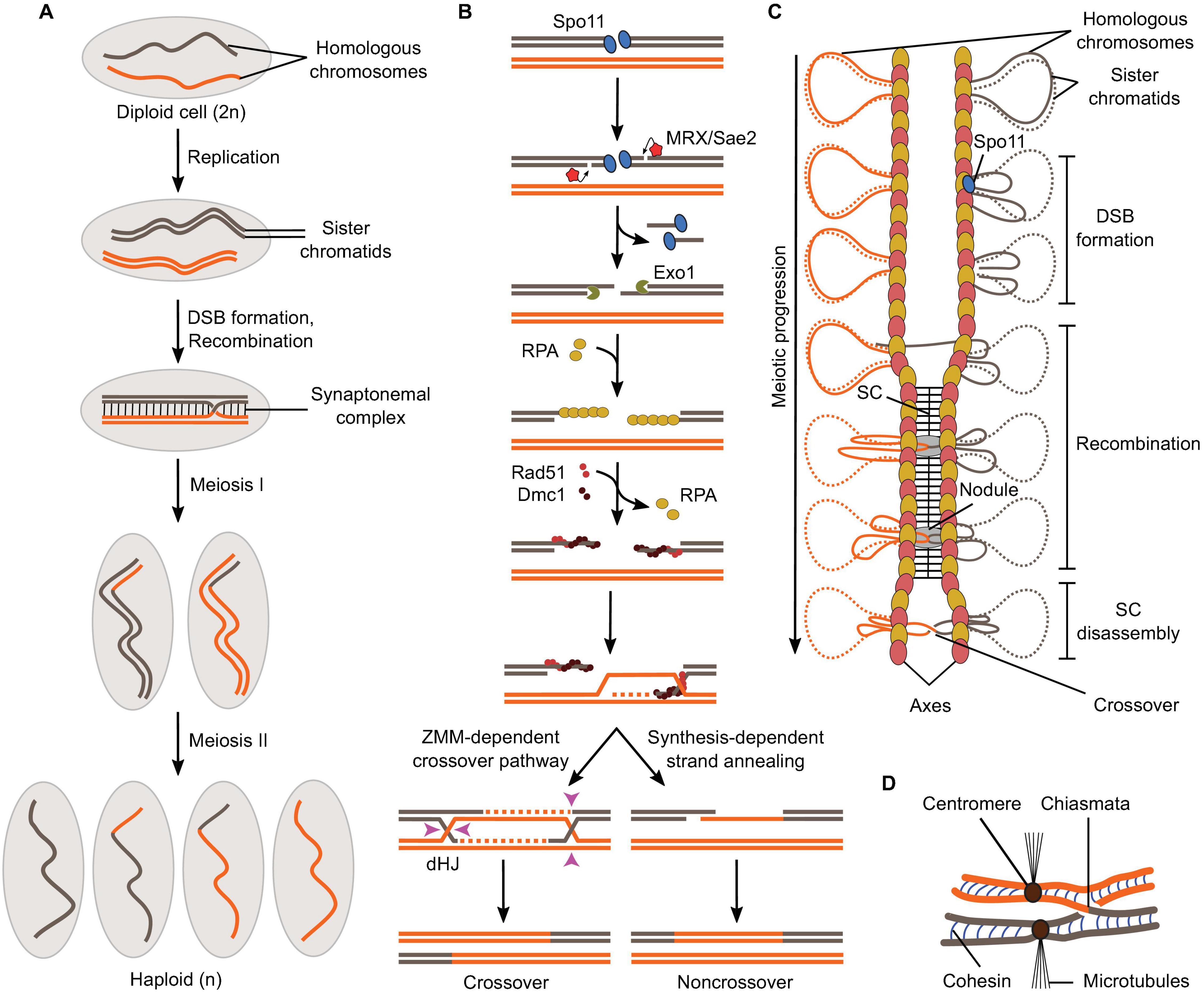This infographic is divided into three distinct panels labeled A, B, and C at the top in bold black letters. The entire graphic is set against a plain white background, providing a clean and clear visual aid without separating lines between the panels. Each panel appears to showcase scientific or medical study data, or possibly a key to various icons.

In panel A, there are wavy lines in black and orange, labeled "homologous chromosomes." An arrow points downward from these wavy lines, labeled "replication to sister chromatids." This panel features double gray and double orange lines extending downward, illustrating the process of replication, with a gray circle accompanying this depiction, providing additional detailed information.

Panels B and C also contain numerous labeled objects with scientific terms or key names, contributing more detailed information. The design and labeling of these elements suggest this infographic is intended to convey complex scientific concepts in a visually accessible manner.